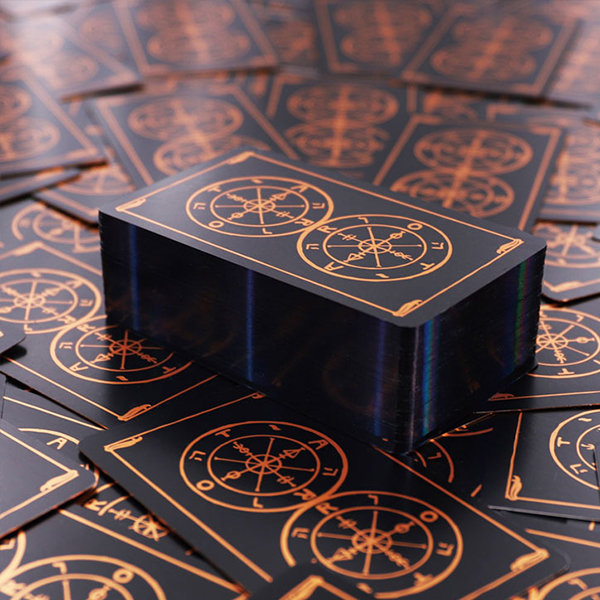This color photograph showcases a collection of intricately designed cards, possibly tarot cards, though no text clarifies their exact purpose. The scene is dominated by a central stack of black cards with glossy black edges. These cards feature detailed gold designs: two concentric circles filled with compass-like lines, arrows, and symbols that resemble zodiac signs, all encompassed by a gold frame. The central stack is surrounded by similar cards scattered beneath it, creating a uniform, radiating pattern. Additionally, a black box with gold trim and lettering is positioned amidst the cards, enhancing the overall dark and mysterious aesthetic. The predominant colors in the image are black and gold, with occasional bronze shading enhancing the depth and richness of the scene.